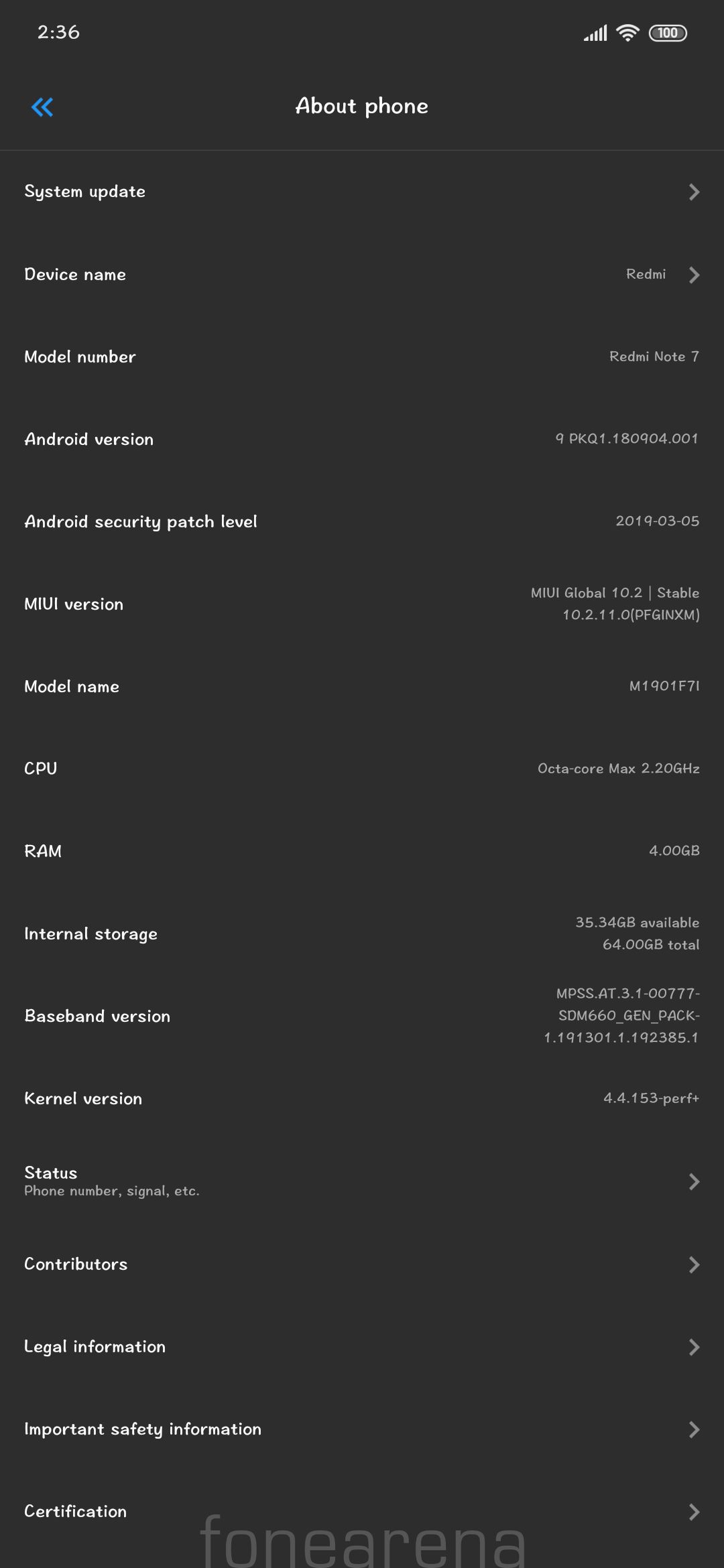The image is a screenshot of an "About Phone" page from an Android device. At the top of the screen, the title "About Phone" is prominently displayed, with a blue back arrow icon located in the top left-hand corner. The arrow consists of two blue lines pointing towards the left.

The black background of the screen indicates that the device is set to dark mode. The text throughout the page is in white, providing clear contrast against the dark background. The page contains an extensive list of information about the phone:

1. System Update
2. Device Name
3. Model Number
4. Android Version
5. Android Security Patch Level
6. Module Name
7. CPU
8. RAM
9. Internal Storage
10. Baseband Version
11. Kernel Version
12. Status
13. Contributors
14. Legal Information
15. Important Safety Information

At the very bottom of the page, in the bottom left-hand corner, there is an entry labeled "Certification." 

Finally, a watermark reading "FONEARENA" (spelled with an 'F') is placed at the bottom center of the screen, subtly indicating the source. This screenshot provides a detailed overview of the various technical specifications and legal information associated with the Android device.